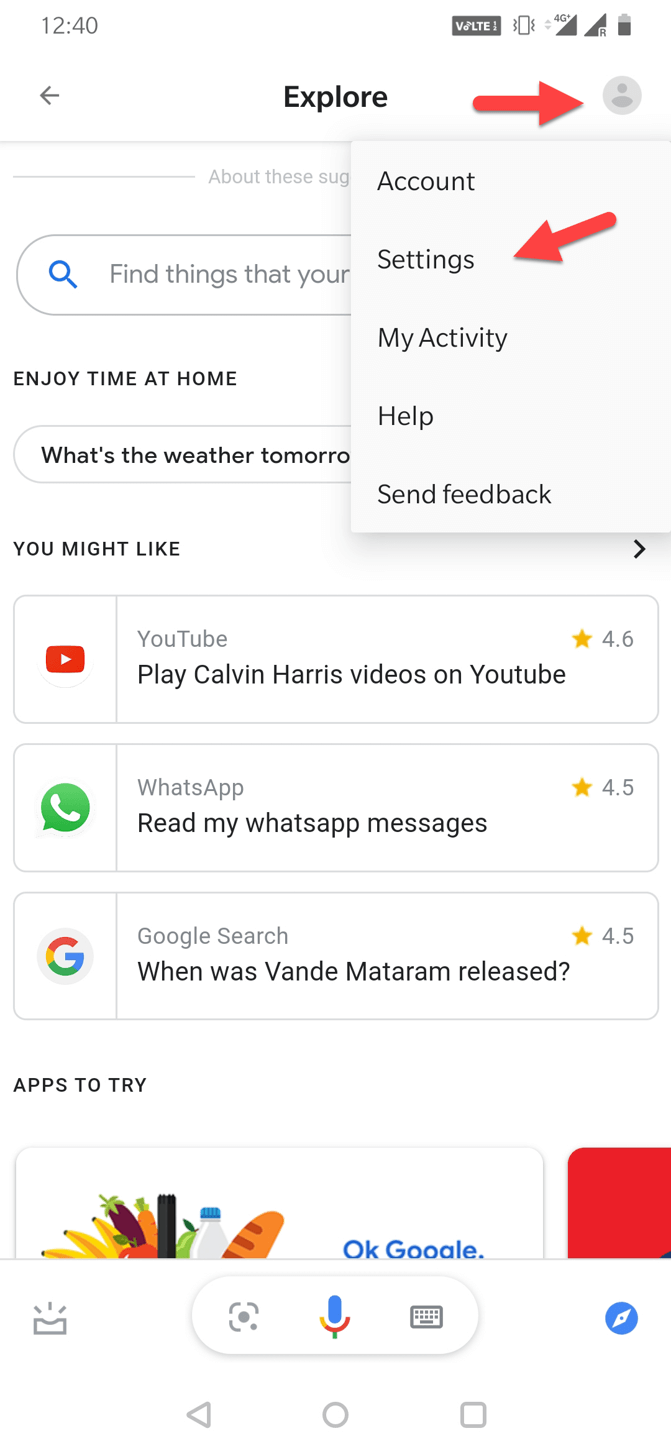The image is a screenshot from a smartphone with a white background. At the very top, the time displayed is 12:40, and to the right of the time, the battery icon indicates it is nearly full. 

Below the time, on the left, there is a back arrow icon, followed by the word "Explore" in the center of the screen. To the right, there is a large red arrow pointing to the account icon. This account icon consists of a circle with an oval shape beneath it. Clicking on this icon reveals a pop-up menu with several options: "Account Settings," "My Activity," "Help," and "Send Feedback." A red arrow specifically points to the "Account Settings" option.

The main portion of the screenshot is a search screen featuring a blue magnifying glass icon. Below the icon, it states, "Enjoy time at home." There is an oval-shaped area with the text, "What is the weather tomorrow?" 

Further down, the screen displays a section titled "You might like," featuring three rectangular recommendation boxes. The first rectangle showcases the YouTube play button with the caption, "YouTube, play Calvin Harris videos on YouTube." The second rectangle has a circular icon with a phone, labeled, "WhatsApp, read my WhatsApp messages." The third rectangle highlights a Google search suggestion, "When was Vandy Matterim released?"